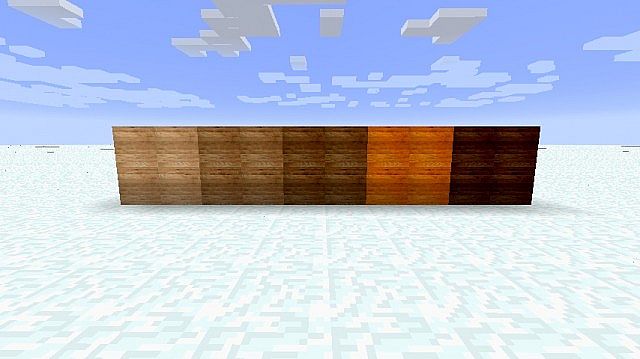The image is a computer-generated drawing that captures a surreal landscape under a blue sky interspersed with clouds shaped like puzzle pieces, rendered in white and shadowed gray hues. At the horizon, a similar puzzle piece motif extends into what appears to be a snow-like surface, predominantly white with tinges of blue. Cutting through the center of the scene is a fence constructed from panels of varying brown shades, evocative of wood grain. The fence features five distinct colors from left to right: light brown, medium brown, dark brown, orangish brown, and very dark brown, all uniformly sized and attached together in a cohesive, yet visually dynamic structure set against the enigmatic backdrop.